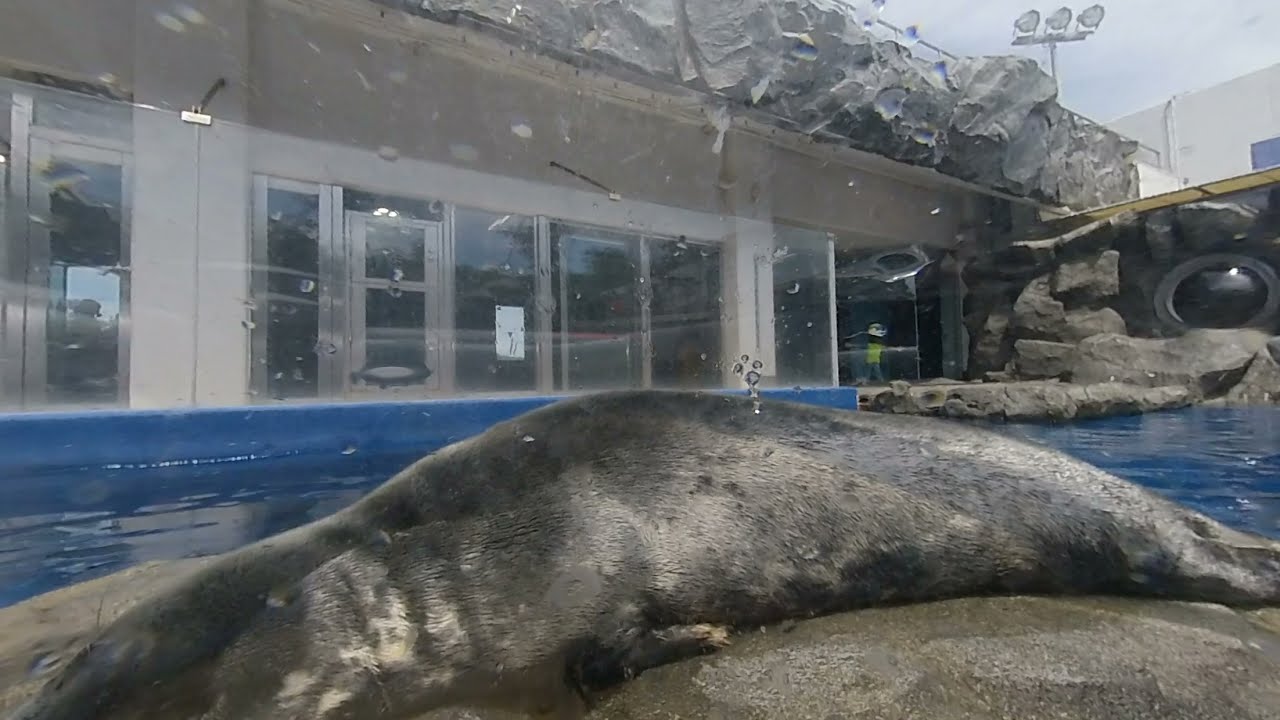This photograph, taken from behind a transparent glass window spotted with water droplets, captures a daytime scene within what appears to be a marine-themed park or aquarium. Central to the image is a large marine mammal, most likely a walrus or seal, resting on a rocky surface within a pool filled with blue water. The animal's black-colored skin is visible, but its full form is partly obscured, making it challenging to identify definitively. The pool area is flanked by artificially created rocks and landmasses. In the background, a horizontally long building with several glass doors and windows is visible, featuring floodlights and a predominantly white facade. The scene is well-lit by natural daylight, highlighting the details and the serene ambiance of the aquatic environment.